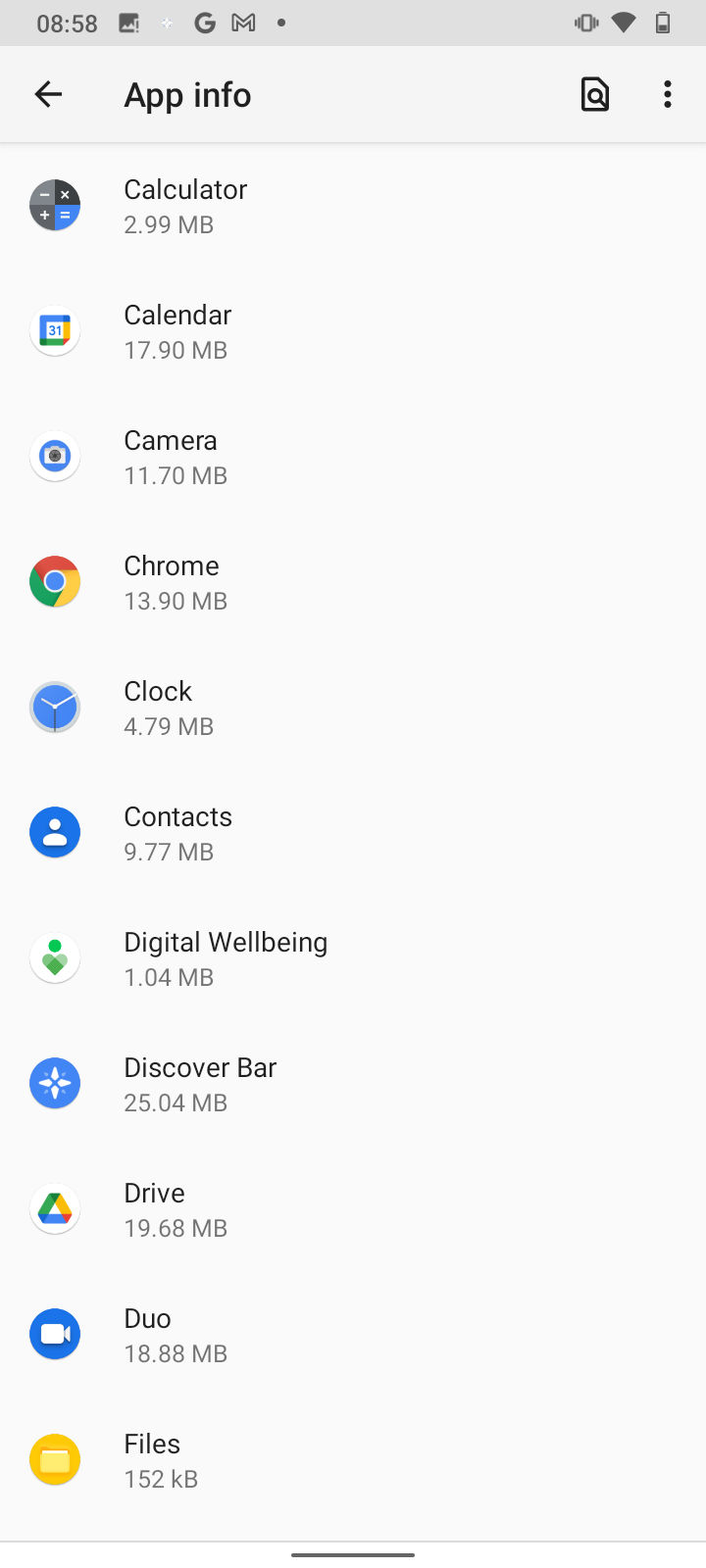Screenshot of a phone screen displaying a list of app options. The screen indicates the time as 8:58 at the top left, alongside icons for a photo, a plus sign, Google, and email (M). Next to these, a vibration signal dot is present, followed by battery meters on the right. Below this top bar is a back arrow and the label "App info." There is a search icon, represented by a magnifying glass, and a three vertical dot menu on the right. A thin gray line separates this section from the list of apps below.

The apps are displayed with good spacing, each accompanied by its colored icon on the left, typical of an Android interface. The apps and their corresponding sizes are listed as follows:
- Calendar (2.99 MB)
- Calendar (17.9 MB)
- Camera (11.7 MB)
- Chrome (13.9 MB)
- Clock (14.79 MB)
- Contacts (9.77 MB)
- Digital Well-Being (1.04 MB)
- Discover Bar (25.04 MB)
- Google Drive, labeled as "Drive" (19.68 MB)
- Duo, the video app (18.88 MB)
- Files (152 KB)

A thin gray line is seen at the bottom of the app list, followed by a shorter, narrower gray line beneath it.